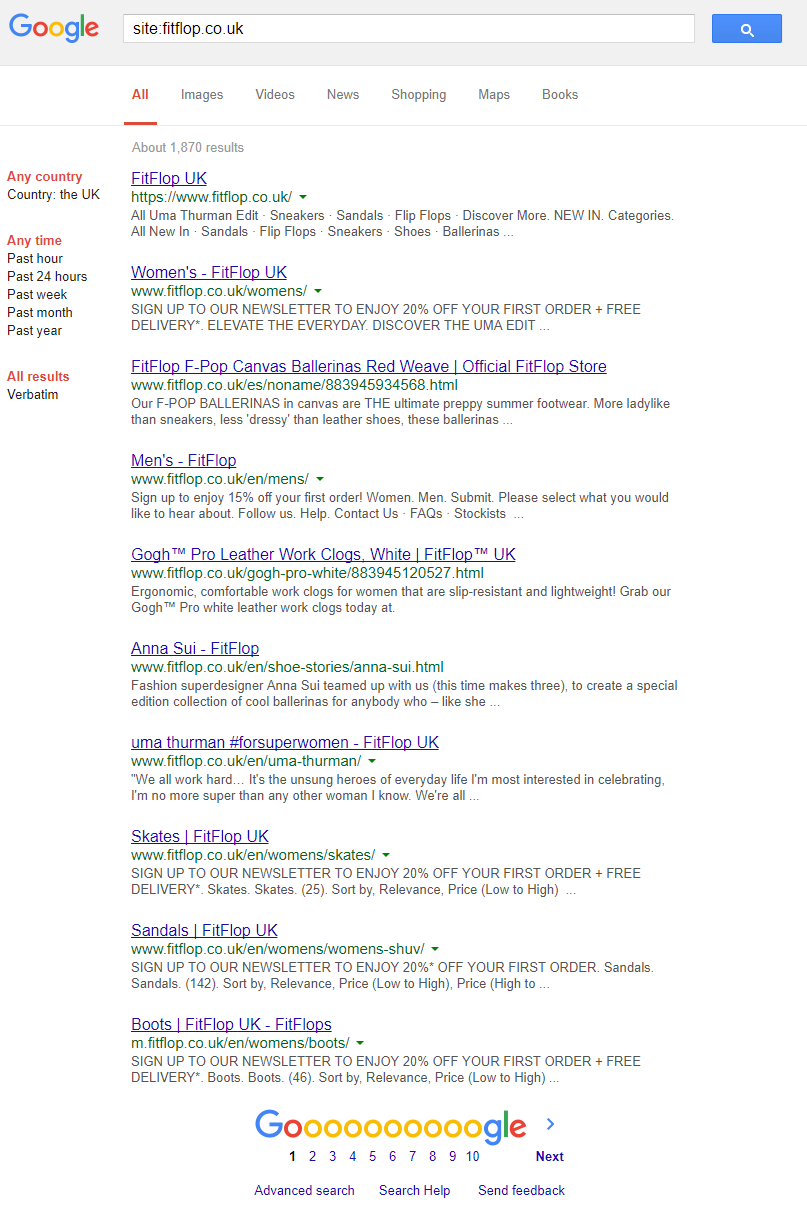A screenshot of the Google.com homepage displays the familiar layout with the Google logo in the upper left corner. Adjacent to this icon is the search field, where "site:Fitflopco.uk" has been entered. To the right of the search bar is the blue search button. Below the search bar, a navigation menu shows options for "All," "Images," "Videos," "News," "Shopping," "Maps," and "Books," with "All" selected and highlighted in red, indicating the current filter. 

The search results reveal 1,870 entries for the query. The visible top ten results include links such as "Fitflop UK," "Women's Fitflop UK," "Fitflop F-Pop Canvas," "Ballerinas Right Weave," and "Official Fitflop Store." To the left, filtering options allow customization by country, currently set to "UK," and time range, with choices from "Past hour" to "Past year."

At the bottom of the screen, pagination options are displayed, showing the first ten pages with a "Next" link to navigate further. The current page is highlighted, indicating that the user is on page 1, with clickable links available to swiftly move to page 2 or beyond.